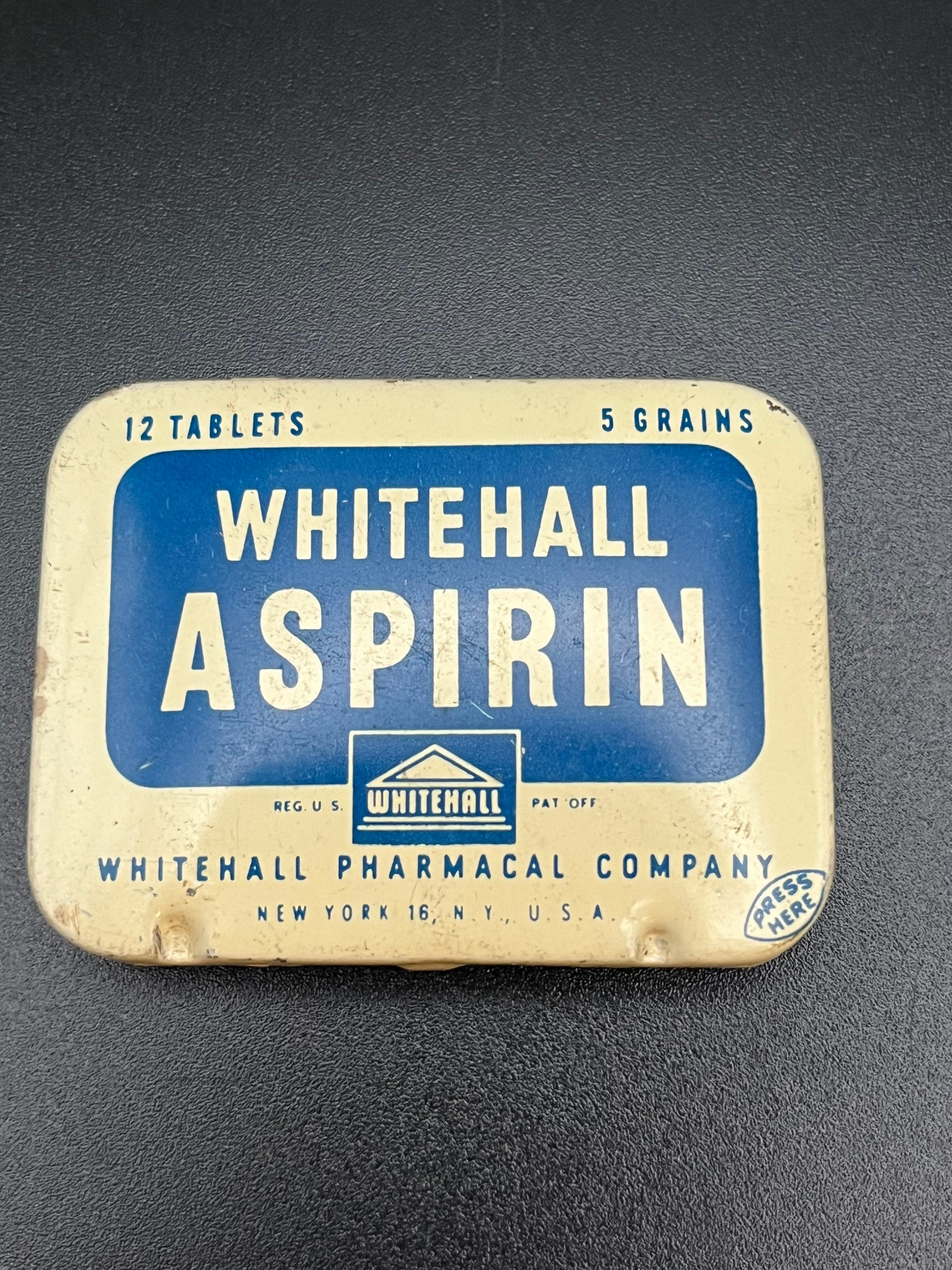This photograph features a vintage tin canister situated on a dark gray or black surface. The canister, likely from the 1930s or 40s, has a metallic sticker with a cream-colored background and a central blue rectangle. Within the blue rectangle, cream-colored text reads "Whitehall Aspirin." Above the rectangle, in the cream area, it states "12 Tablets" at the top left and "5 Grains" at the top right. Below the rectangle, additional blue text reads "Whitehall Pharmacal Company, New York 16, NY, USA." The words "Reg US Pat Off" appear under the central label. In the bottom right corner, the sticker contains the instruction "Press Here" in a diagonal orientation, likely indicating how to open the canister. The overall vintage and aged appearance of the tin, along with the detailed labeling, emphasize its historical and collectible nature.